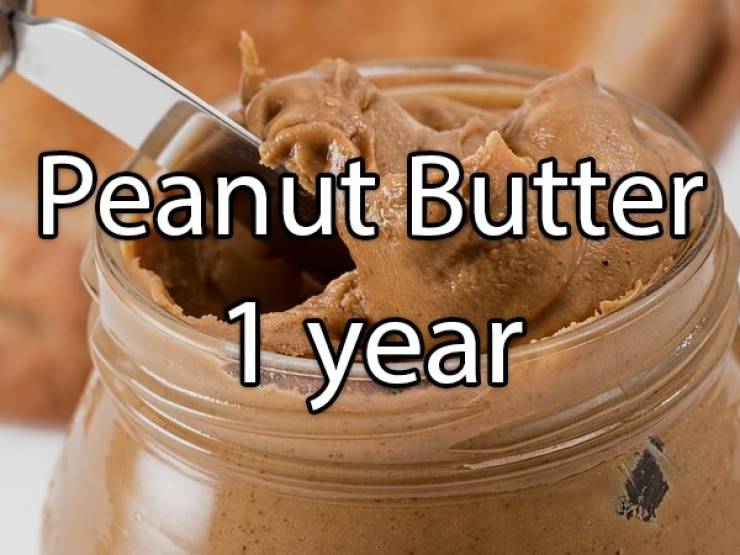The image is a close-up of an opened, mostly full jar of brownish, smooth-textured peanut butter. A silver, reflective butter knife is seen digging into the top-left area of the peanut butter, poised to scoop some out. The jar, which is made of clear glass, occupies the majority of the frame, with the visible portion being about 2 to 3 inches high. The screw lid has been removed and is not visible in the picture. White text with a black outline is superimposed in the center of the image, reading "peanut butter" on the first line and "one year" on the second line. The background is blurred and predominantly brown, with indistinguishable objects that could be a piece of toast or another peanut butter jar. Some portions of what might be counter space are barely visible in the lower left and upper right corners of the photo.